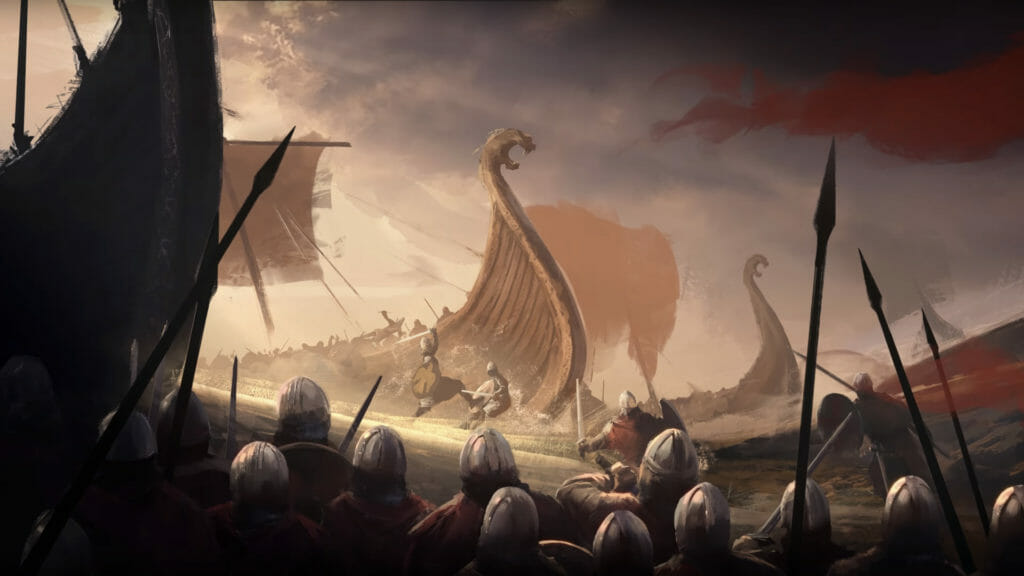In this detailed painting of a dramatic Viking scene, dark and ominous gray clouds fill the sky, creating an intense backdrop for the action below. Flashes of white and blue light, along with portions of red smoke and fire, further enhance the chaotic atmosphere. Central to the composition are several wooden Viking ships, characterized by their brown hues and intricate dragon head prows that rise impressively from their decks. 

On one of these ships, a group of armored Viking warriors, distinguishable by their helmets and carrying swords and spears, are depicted. A large sail dominates this vessel, hinting at the wind and turmoil at sea. To the left, a massive spear points upwards, emphasizing the anticipation of imminent battle.

On the ground, another group of Viking soldiers stands ready for combat, their intent to confront those arriving from the ships clear in their poised spears and determined stances. The scene suggests a fierce and impending clash, with the soldiers on land seemingly prepared to attack their seafaring counterparts. This vivid and adrenaline-pumping depiction offers no information on its artist or origin, but it vividly captures a moment steeped in historical and mythological vigor.